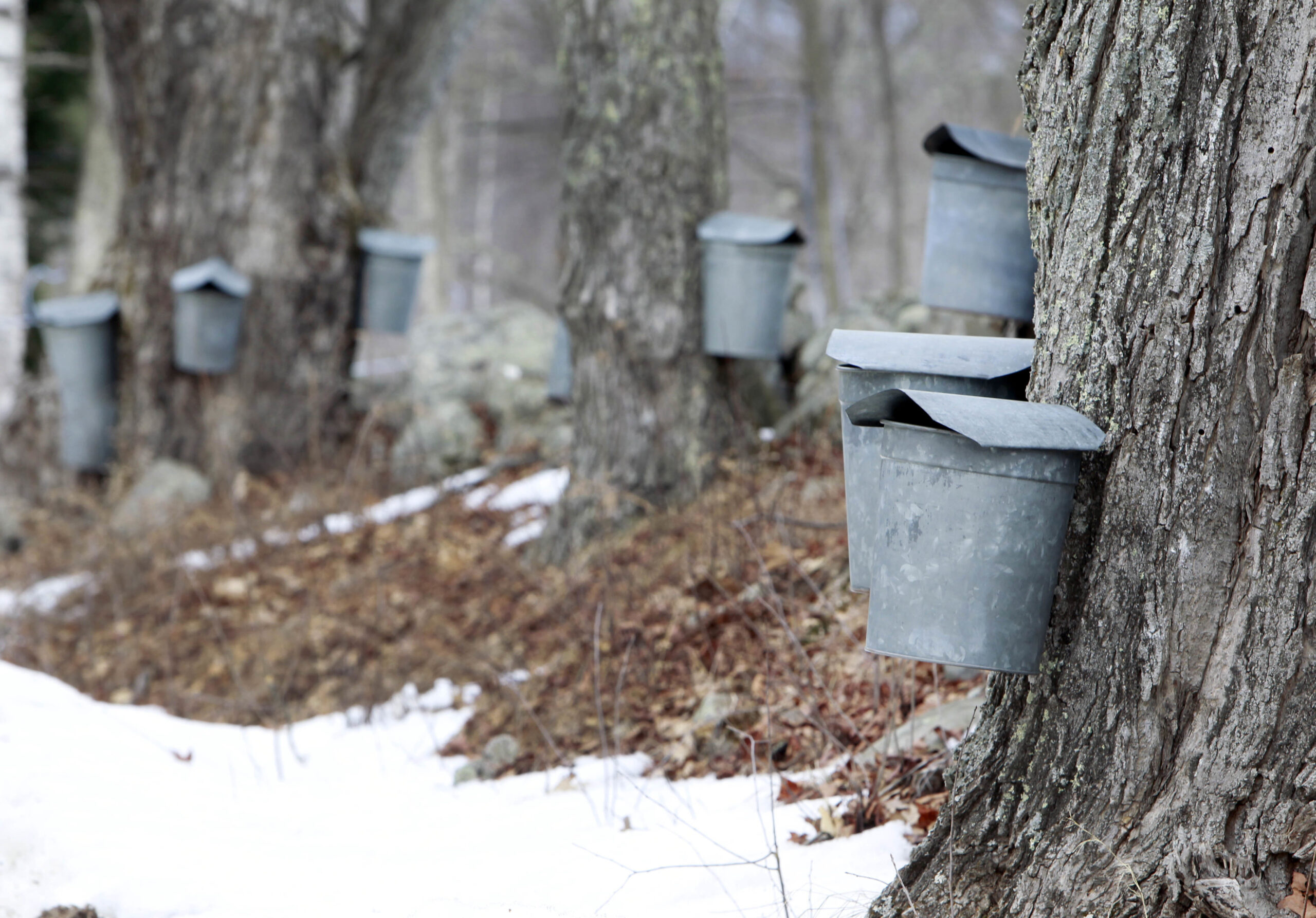A picturesque forest scene captures a serene winter landscape where maple trees are being tapped for their precious sap. The foreground features a blanket of pristine white snow, tapering off towards the right-hand side where a prominent tree trunk stands. Silver buckets are affixed to each maple tree with small, glinting tin spouts carefully inserted into the bark to collect the sap. Nine buckets can be counted, arrayed throughout the scene, with the front two in sharp focus while the rest gradually blur into the background, indicating a shallow depth of field. The forest floor is scattered with brown leaves and underbrush, hinting at the late autumn or early winter setting, possibly in Vermont. The background remains softly out of focus, adding an intimate, macro feel to the image and emphasizing the tactile details of the process and the tranquility of the woodland setting.